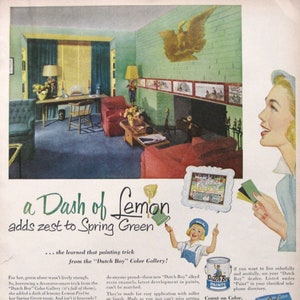The advertisement, likely from a 1940s or 50s magazine or newspaper, vividly portrays a vintage living room adorned with a green brick wall on the right and a cozy fireplace. The floor is covered in blue carpet, and the room is furnished with red chairs and illuminated by various lamps. A window with yellow curtains adds a touch of brightness to the mint-green walls, echoing the ad's tagline, "A dash of lemon adds zest to spring green." 

In the foreground, a cheerful figure in blue overalls and a blue hat, holding a paintbrush, points upward, seemingly admiring the room's fresh look. To the right, a blonde woman gazes up at the room, her expression suggesting admiration or contemplation. She holds an indistinct object, possibly money, implying she's considering a purchase related to the room's decor. The bottom of the ad mentions "the Dash and Bay Color Gallery," hinting that the green and yellow tones are featured paint colors available for purchase.